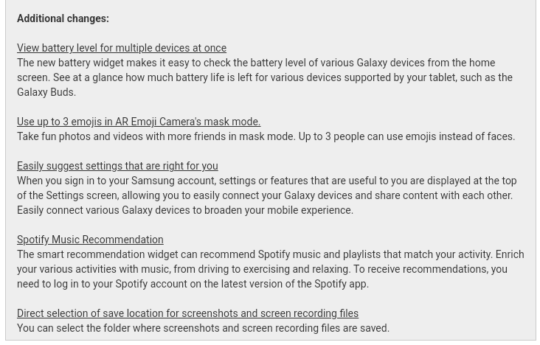**Detailed Screenshot Description:**

The image is a screenshot featuring a gray background with black and gray text, titled "Additional Changes." Below the title, there are five underlined categories, each with its own detailed description.

1. **View battery level for multiple devices at once**: This section explains the functionality of the new battery widget, which allows users to monitor the battery levels of various Galaxy devices directly from the home screen. It mentions that users can easily check the remaining battery life of devices like the Galaxy Buds supported by their tablet.

2. **Use up to three emojis in AR Emoji Camera's mask mode**: This category describes a feature in the AR Emoji Camera's mask mode where up to three users can replace their faces with emojis to take fun photos and videos. It emphasizes the social aspect of this functionality.

3. **Easily suggest settings that are right for you**: Upon signing into a Samsung account, users are presented with personalized settings or features at the top of the settings screen. This facilitates effortless connection and content sharing between multiple Galaxy devices, thereby enhancing the mobile experience.

4. **Spotify music recommendation**: The smart recommendation widget suggests Spotify music and playlists tailored to users' activities like driving, exercising, or relaxing. It requires users to log in to their Spotify account on the latest app version to receive these personalized recommendations.

5. **Direct selection of save location for screenshots and screen recording files**: This feature enables users to choose the specific folder where their screenshots and screen recording files are saved, providing more control over file organization.

The image features a clear, easy-to-read font with no additional content, making the information straightforward and accessible.